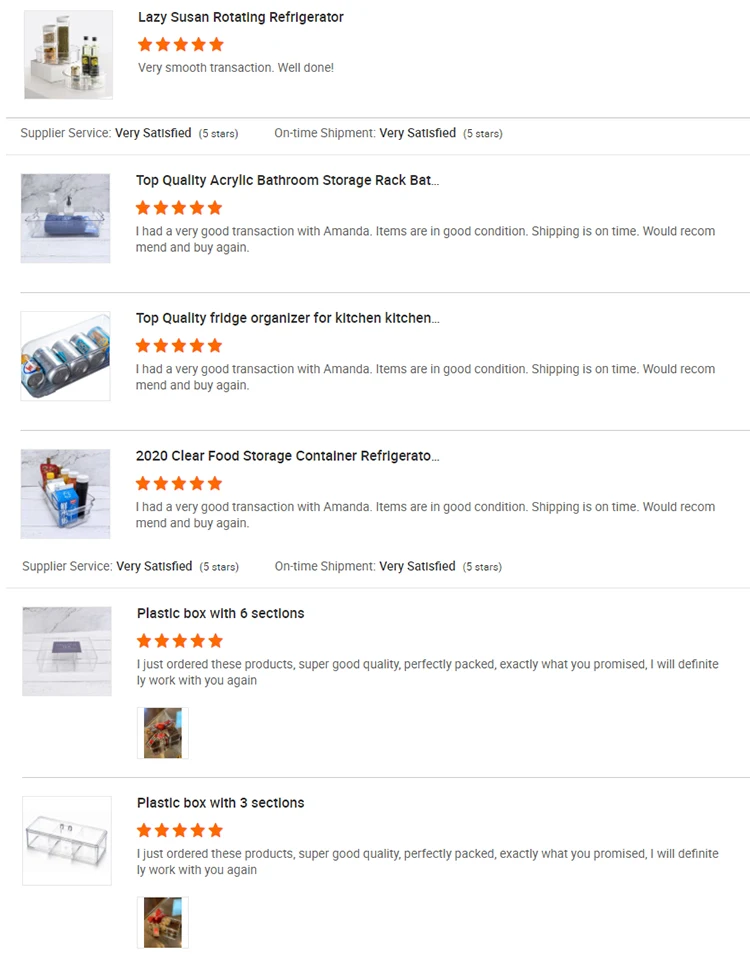The image showcases reviews of six different products arranged in a two-column layout on a white background. On the left side of the image, there are pictures of the products, each accompanied by the product name on the right. The top product is a Lazy Susan rotating refrigerator, which has received a five-star review praising the transaction as "very very smooth" and commending the job as "well done." All products on this image have received five-star ratings, with the stars depicted in orange. The last two products at the bottom have accompanying photos below their reviews. The review for the bottom-most product, a plastic box with three sections, highlights its super good quality, perfect packaging, and fulfillment of promises, concluding with a commitment to future collaborations. The product names are displayed in black for easy readability.